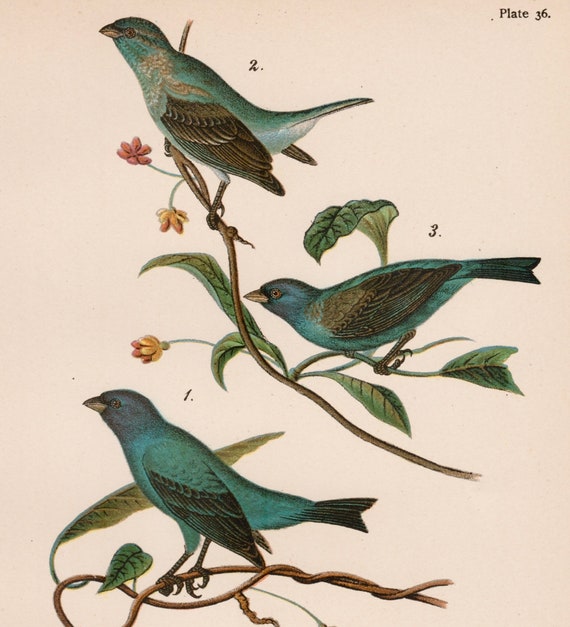This illustration, titled "Plate 36" and taken from a book of bird drawings, features three colorful finches perched on vine-covered branches adorned with small orange-red flowers. The birds are labeled one, two, and three and exhibit varying plumage. The first finch, at the bottom left, showcases a bluish-teal body and a bluish head, with wings tinged in brown and a short, slightly sharp beak. The second finch, positioned at the top, has a predominantly turquoise or blue-green body with black wings and a distinctive silver plumage along its neck. It also sports lighter blue tail feathers and a dark orange beak. The third finch mirrors the first in coloration with its green-blue body, brown wings, and a beige beak. All the birds feature a vivid yellow eye with a black pupil and are artistically captured standing on different sections of the viney branches.